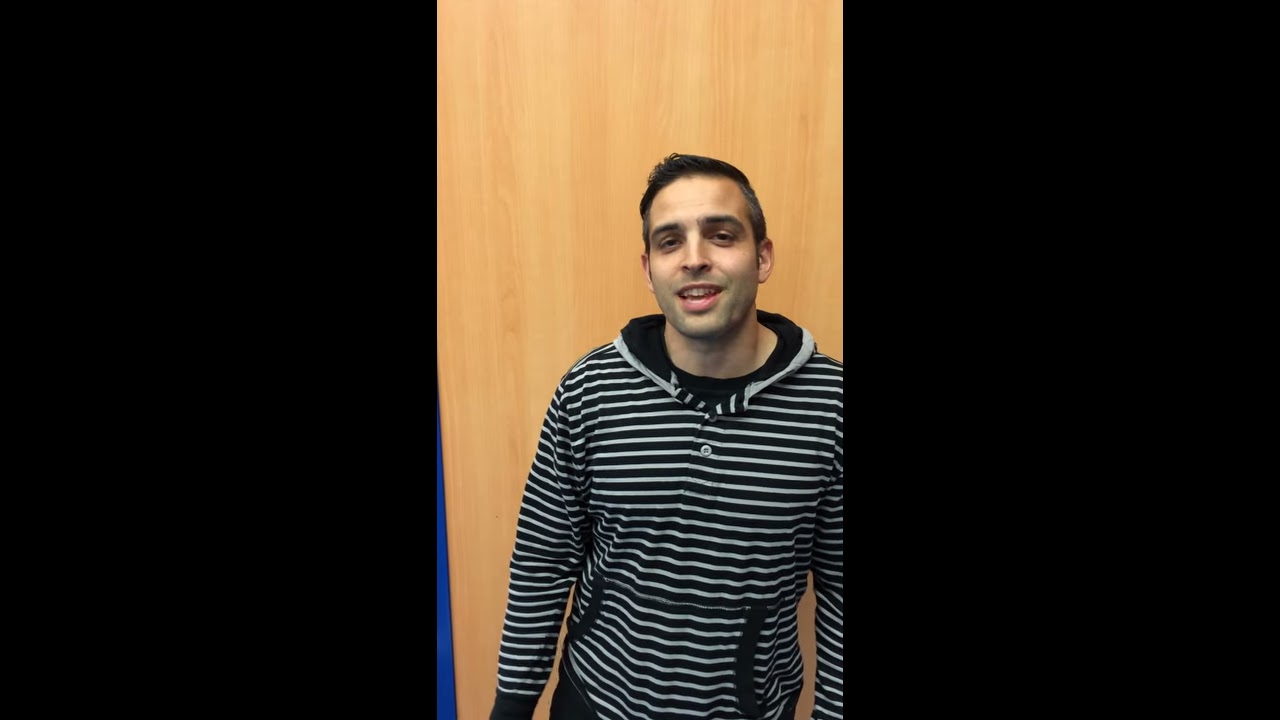This photograph features a young man, likely in his late 20s or early 30s, standing in front of a wooden door or a wooden panel wall. He has short dark hair and bushy eyebrows, with an olive or caramel complexion. He is wearing a black and gray striped hoodie with a front kangaroo pocket and a button near the chest area. The inside of the hoodie is black. The man is smiling at the camera with slightly squinted eyes, possibly as if caught mid-sentence or posing for a new profile picture. It is a vertical, rectangular photo that focuses solely on him, with no additional elements in the background.